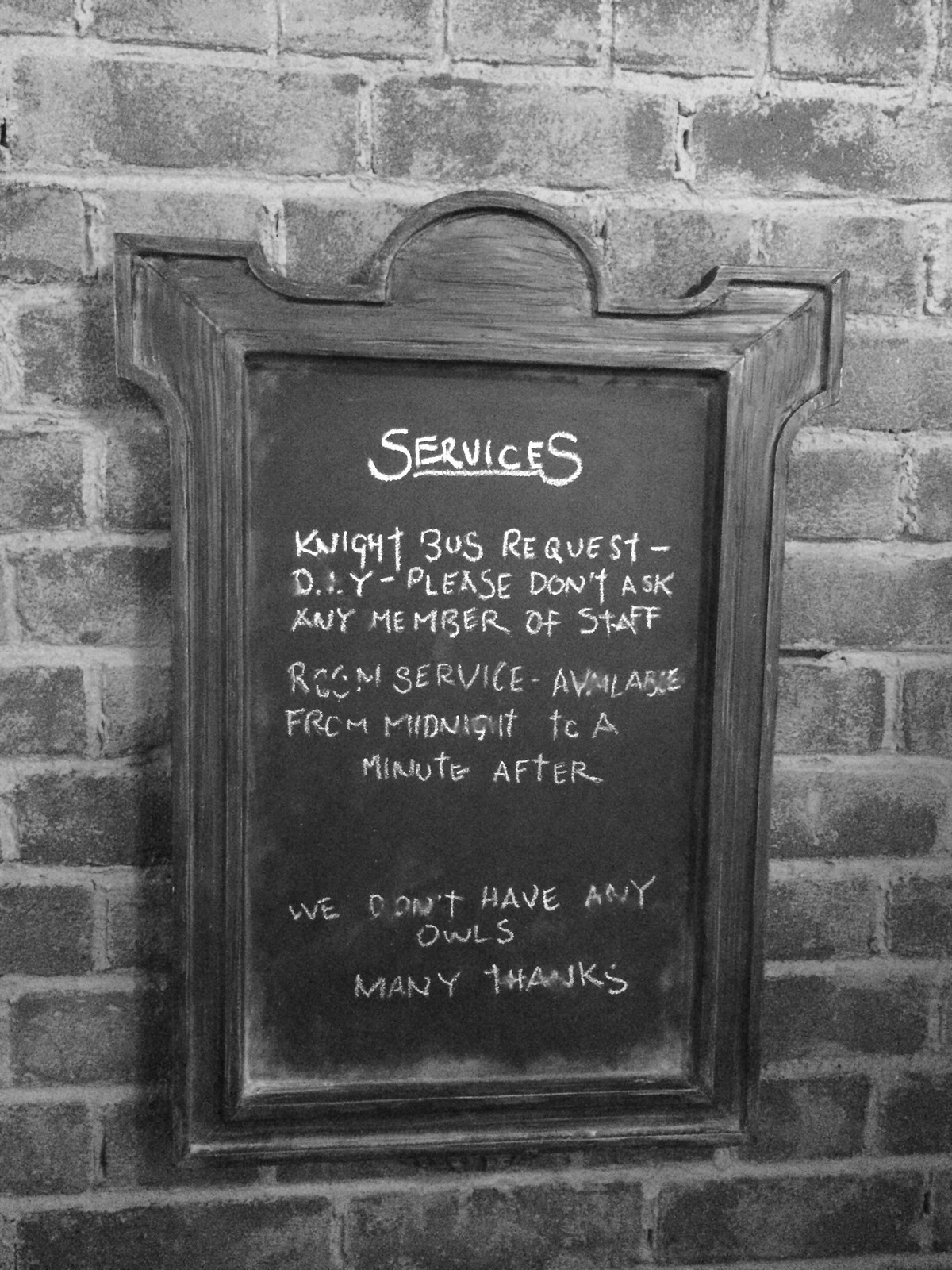In this black-and-white photograph, we see a creatively designed chalkboard sign mounted on a large brick wall. The chalkboard, framed in intricately carved wood with elegant arches and pointed tops, serves as an eye-catching announcement plaque. Written in white chalk, though a bit smudged, the sign reads "Services," which is underlined at the top. Below, the text lists several whimsical statements: "Night Bus Request, DIY, Please Don't Ask Any Member of Staff, Room Service Available from Midnight to a Minute After, We Don't Have Any Owls, Many Thanks." These playful messages evoke a sense of charm and are reminiscent of themes from the Harry Potter series.